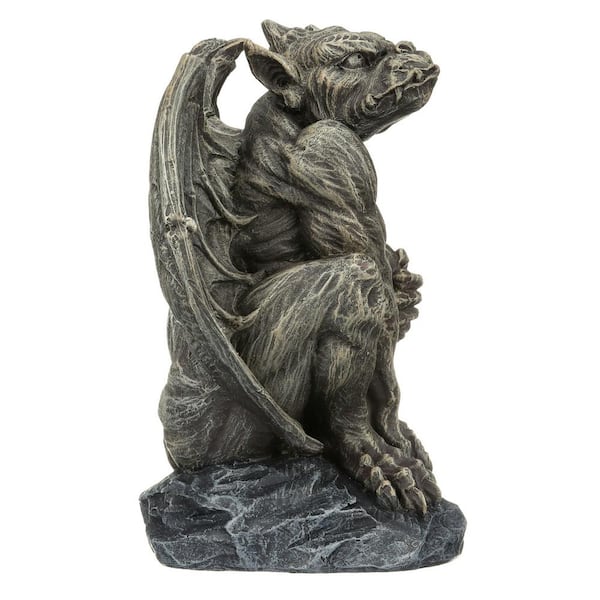This detailed carved statue depicts a muscular gargoyle-like creature perched on a dark gray, rock-textured base. The gargoyle, striking an imposing figure, has prominent pointed ears, fangs protruding from its mouth, and large wings folded against its back. Its stone gray hue is interspersed with blue tones and white veining that add depth to its appearance, while subtle yellowing enhances the rugged, earthy texture. The creature appears to be gripping its chest, possibly suggesting an injury, while its stern, grotesque face gazes upwards as if anticipating something. The overall image captures a blend of gothic and mythical elements, embodying a sense of foreboding and strength.